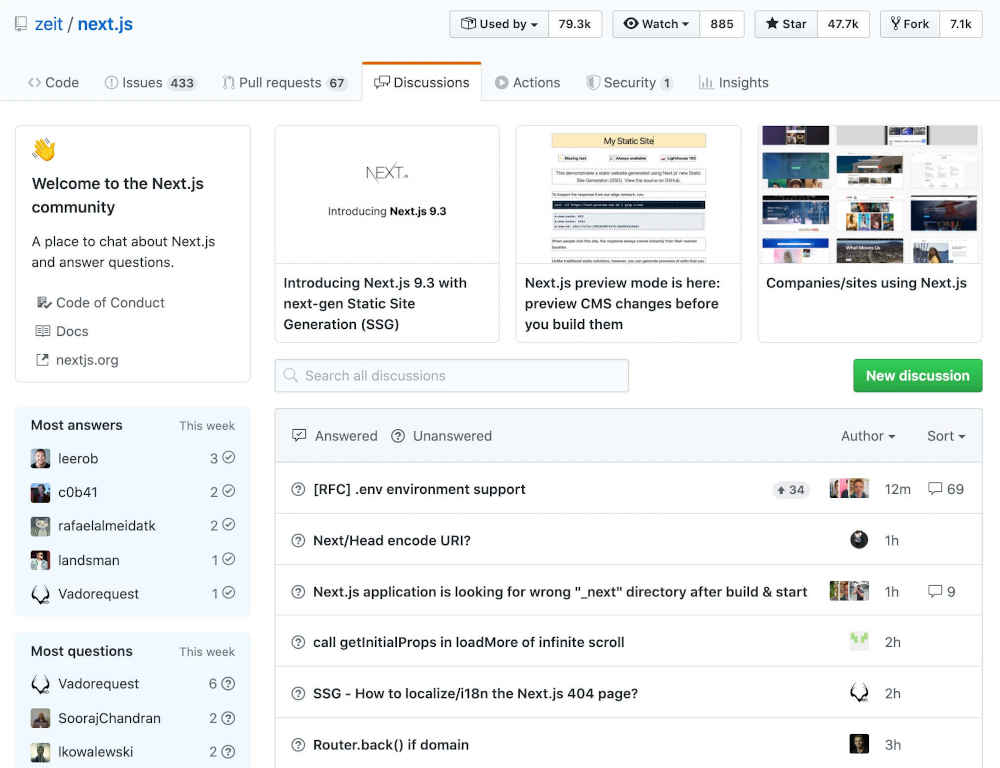Screenshot of the Next.js Message Board on ZEIT

The image is a screenshot of the Next.js message board on the ZEIT website, resembling a forum similar to Reddit. On the left side of the interface, there are vertical bars indicating the top users based on the number of answers and questions they have posted. To the right, there is a forum-style listing of answered questions. Each question is displayed with the author's name, which is clickable, allowing users to view submitted answers. At the very top of the page, a horizontal menu provides navigational submenus labeled 'Code,' 'Issues,' 'Pull Requests,' 'Discussions,' 'Actions,' 'Security,' and 'Insights.'